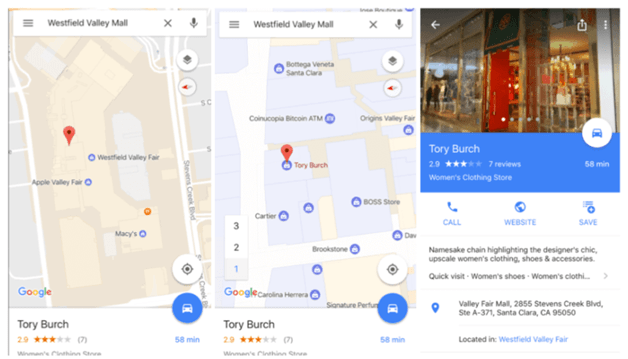Here is an improved and detailed caption for the described image:

"The image consists of a series of three cell phone screenshots taken at different times throughout the day, all focusing on the Westfield Valley Mall. The leftmost screenshot displays a map of the mall with a highlighted red dot indicating the location of the Tory Burch store. This initial map provides a general overview of the mall's layout, including various shops and pathways.

The second screenshot, adjacent to the first, zooms in on a more specific section of the mall. It offers a closer view of the Tory Burch store's precise location within the mall, helping users to navigate directly to the store.

The third and final screenshot features an image of the Tory Burch store itself, accompanied by review information. The reviews are notably poor, suggesting that the store is not highly rated by customers. Additionally, the screenshot provides contact information and a link to the store’s website for further details.

Together, these screenshots effectively guide the viewer from a broad overview of the mall to a focused image of the Tory Burch store, along with pertinent review and contact information."